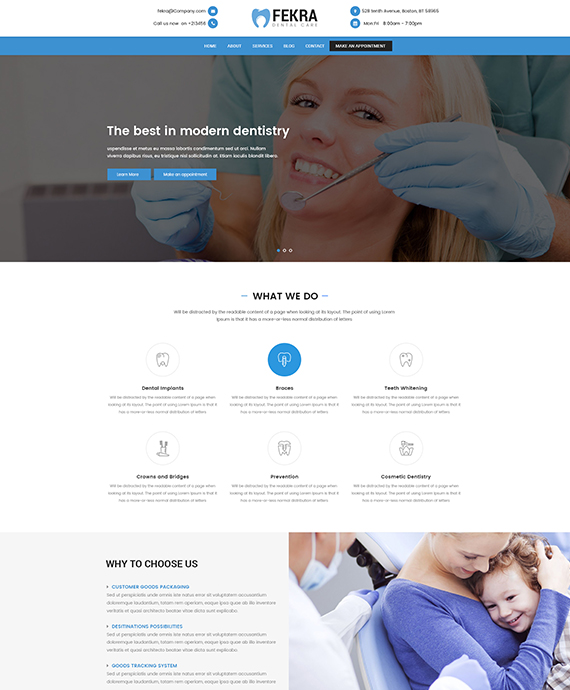**Detailed Caption:**

The screenshot captures the homepage of FECRA Dental Care's website, set against a pristine white background. At the top left corner, contact details including an email address and telephone number are prominently displayed alongside respective icons for easy identification. Centrally positioned is the FECRA Dental Care logo, featuring ‘FECRA’ in bold black letters and ‘Dental Care’ below it in a lighter black font, accompanied by a distinctive blue tooth icon. To the left of the logo, the address is clearly listed, while the clinic hours are conveniently located to the right.

Beneath this header section, a large blue banner spans the width of the page, presenting various categories related to dental services. Positioned towards the right end of the banner is a conspicuous black button inviting visitors to "Get an Appointment."

Dominating the main body of the webpage is a welcoming image of a woman seated comfortably in a dental chair, smiling broadly as a dental professional, clad in a blue smock and plastic gloves, holds a dental mirror up to her mouth. This professional is likely a dentist or dental hygienist, enhancing the image of a friendly and professional environment.

Directly below this image, the section titled "What We Do" features several icons, each accompanied by a brief description of services offered. 

At the bottom of the webpage, the "Why Choose Us" section provides additional reassurance to potential clients, showcasing a large image on the right and a series of bullet points highlighting reasons to opt for this dental practice.